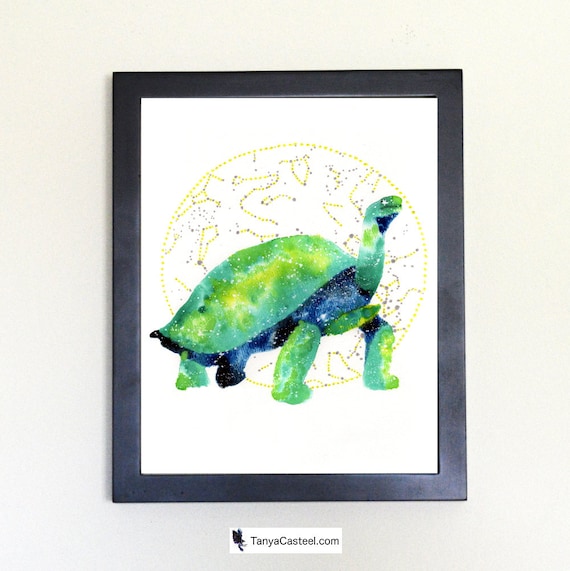This detailed watercolor painting by Tanya Castiel, displayed on tanyacastiel.com, features a vividly colored turtle set against a celestial backdrop. The artwork is encased in a black frame approximately an inch thick, which surrounds a white canvas. At the center of the painting, a turtle with a lively blend of greens, yellows, and blues stands upright, its neck extended and head turned towards the upper right. The shell and limbs exhibit varying shades of green and yellow, while the underside transitions into a blue hue with hints of dark blue and black.

Behind the turtle, a large dotted circle dominated by yellow outlines suggests a constellation-filled night sky. The constellations are intricately depicted with fine lines, appearing as ethereal patterns scattered throughout the background. The overall image exudes a surreal, almost floating quality, as the turtle seems suspended in mid-air, surrounded by this magical starlit scenery. The painting merges the earthy elements of the turtle with the otherworldly aura of the cosmos, creating a captivating and harmonious visual masterpiece.